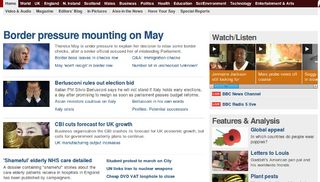The image, sourced from a website, showcases a chaotic array of news articles, headlines, and multimedia content. Dominating the visual top is the headline "Border Pressure Mounting on May," accompanied by three distinct images: a woman, a politician with hands over his face, and another woman wearing a mask. Towards the bottom of the image, a headline reads "CBI Cuts Forecast for UK Growth," under which appears "Rules Out Election Bid" with a partially obscured politician's name due to the image's blurriness. The left side features an assortment of articles and links, though the text is difficult to decipher. On the right, there are options to watch and listen to three different videos, plus additional features and in-depth analysis, including a segment titled "Low Letters to Low Voice" or possibly "Louie." The overall layout is busy, reflecting a mixture of news, analysis, and multimedia elements aimed at providing a comprehensive news experience.